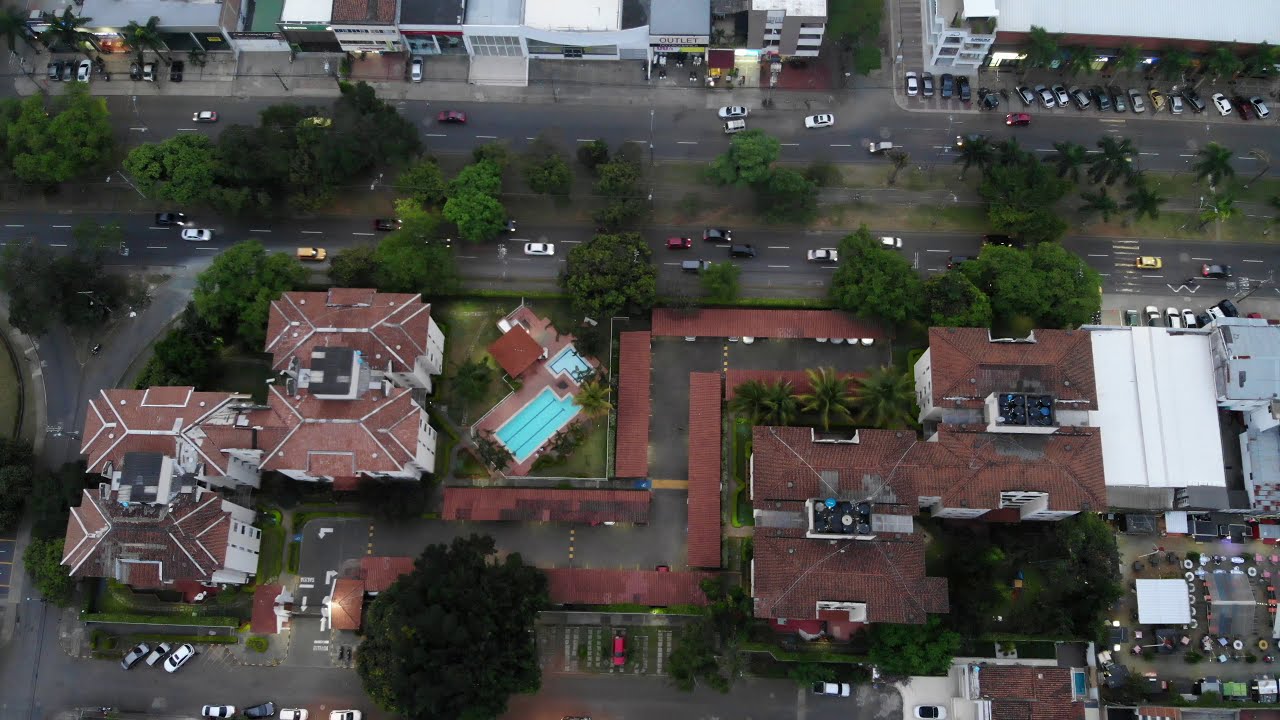An aerial view of a city reveals a bustling residential and commercial area intersected by a highway. In the bottom left corner, two multi-story buildings with white walls and orange-tiled arched roofs stand prominently. Adjacent to these buildings is a light green swimming pool with three lanes, accompanied by what appears to be a smaller sauna pool. A concrete pathway weaves away from this cluster towards the right, curves upwards, and continues to another set of buildings with similarly styled but slightly dirtier orange-tiled roofs. In close proximity, a building with a white roof can be seen.

Beyond this concentration of structures lies a murky street heading left and right, lined with numerous cars both in motion and parked. The central divider of the road is lush with grass and an assortment of dark to light green trees. The dreary atmosphere suggests recent rainfall, contributing to the dirty and wet appearance of the roads and rooftops. Towards the top, various storefronts and commercial buildings are visible, with a notable sign for an "outlet" in the midst. The image showcases a clear distinction between the residential complexes on one side and the commercial area on the other, highlighting a well-populated urban locale brimming with activity and vehicles.